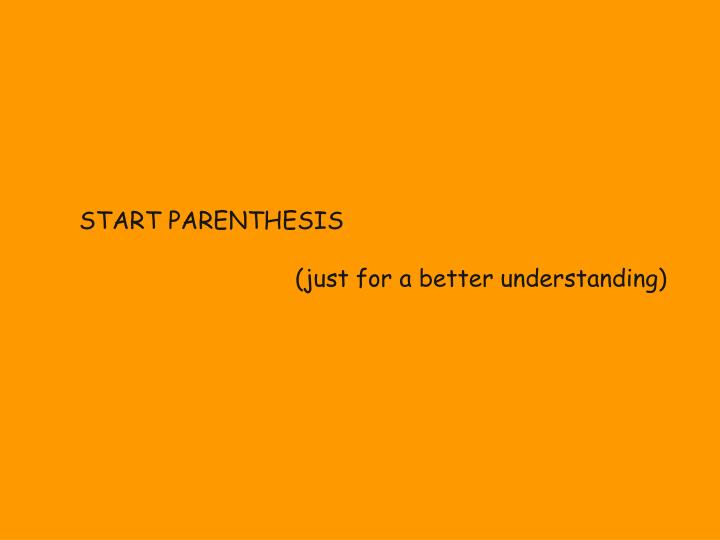The image is a minimalist graphic with a solid orange background occupying the entire landscape-oriented rectangle. The only content is black text in Comic Sans font. In the upper left quadrant, the text reads "START PARENTHESES" in all caps. Positioned just below and slightly to the right of this, in lowercase within parentheses, it reads "just for a better understanding." The orange backdrop and the monocolored text create a clean, straightforward visual style. The words are aligned such that "START PARENTHESES" is more to the left and "just for a better understanding" is offset to the right, maintaining balance without being perfectly centered.